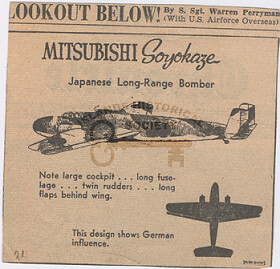This detailed image is a black and white newspaper clipping, possibly from the 1940s during World War II. It features an article by Sergeant Warren Perryman with the U.S. Air Force Overseas titled "Look Out Below!" prominently displayed in gray with an exclamation point. The main focus of the clipping is an advertisement or alert about the Mitsubishi Soyokaze, a Japanese long-range bomber. The article includes a detailed graphic image of the airplane, highlighting key features such as its large cockpit, long fuselage, twin rudders, and lengthy flaps behind the wings. Additionally, there's a drawing on the right side of the clipping that depicts another view of the plane, emphasizing German influence in its design. The newspaper has a faded, beige hue, indicative of its age, with ink bleeding through from the other side, adding to the historical authenticity of the piece.